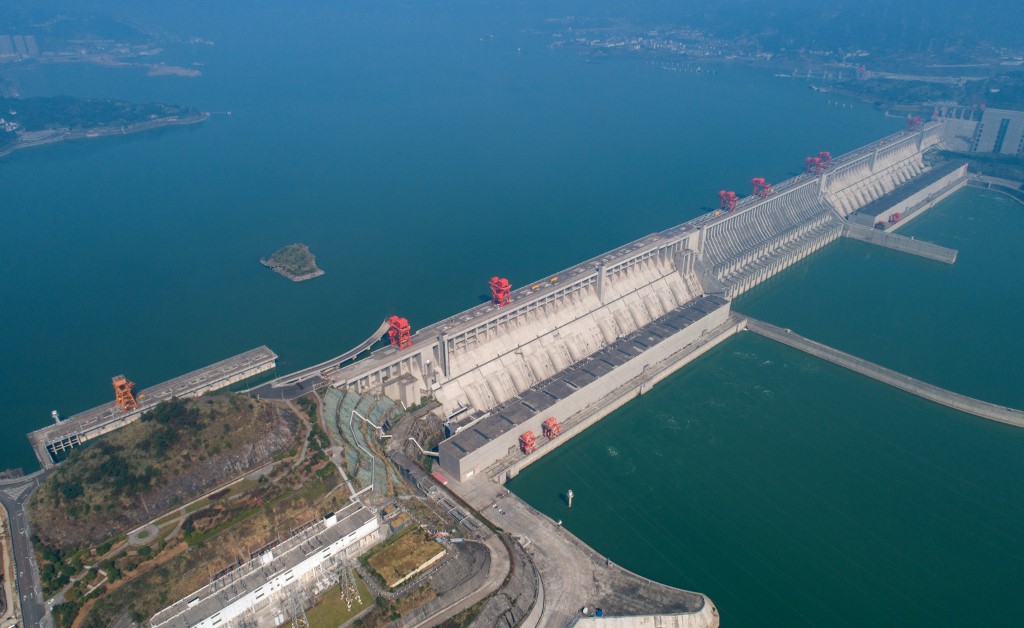This detailed aerial photograph, taken from a great height, depicts a massive concrete dam spanning a broad, bluish-green river. The dam divides the river into two distinct areas and features various sections with locks and drainage points. On top of the dam, there is a bridge bustling with heavy traffic, with cars traveling in both directions. Adding to the complexity, a row of red structures, likely pumps or supports, lines the top of the dam. In the lower left corner, a rock outcropping with vegetation suggests that part of a mountain was blasted away to construct the dam. The image also shows a couple of small islands dotting the river and stretches of land on either side, contributing to the intricate landscape.